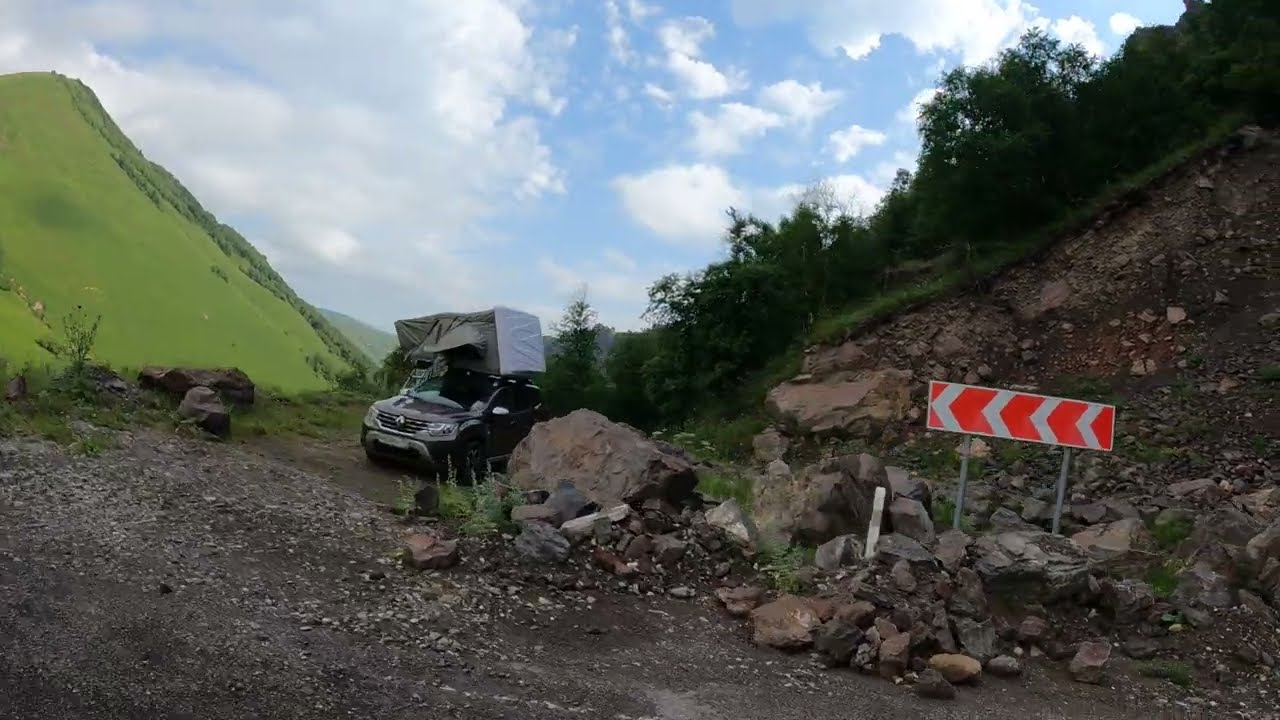In this outdoor daytime scene, a black compact SUV is parked in the middle of a rocky, valley-like area surrounded by large boulders and gravel. The vehicle has a gray, tent-like structure or cargo load on top of it. Positioned towards the right side of the scene, an orange road marking sign with white arrows points leftwards towards the vehicle, suggesting it might have missed a turn. The landscape includes a bright lime green, grassy hill to the left and a lush, shrubbery-filled hill to the right, forming a V-shape. In the distance, a blue sky with fluffy clouds stretches across the horizon.